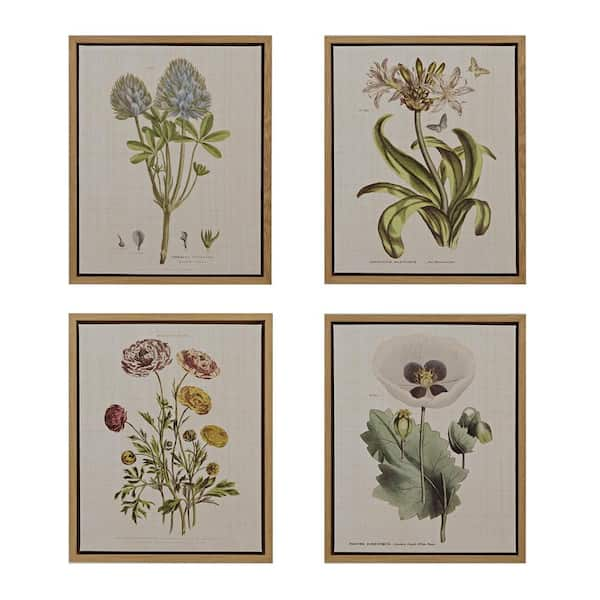This photograph showcases a two-by-two grid of framed paintings, each depicting a unique flower. All four pieces are surrounded by tan wooden frames. In the upper left corner, the artwork features a blue, fuzzy, cluster-like flower with abundant green foliage. Adjacent to it, in the upper right corner, is an illustration of a white flower with long, green leaves. The lower left corner portrays a bouquet of disc-shaped flowers, combining hues of purple, yellow, and red on a single plant, reminiscent of carnations. Lastly, the lower right corner displays a white pansy with subtle purple markings. The overall composition highlights an array of colorful blossoms, each intricately detailed in their respective frames.